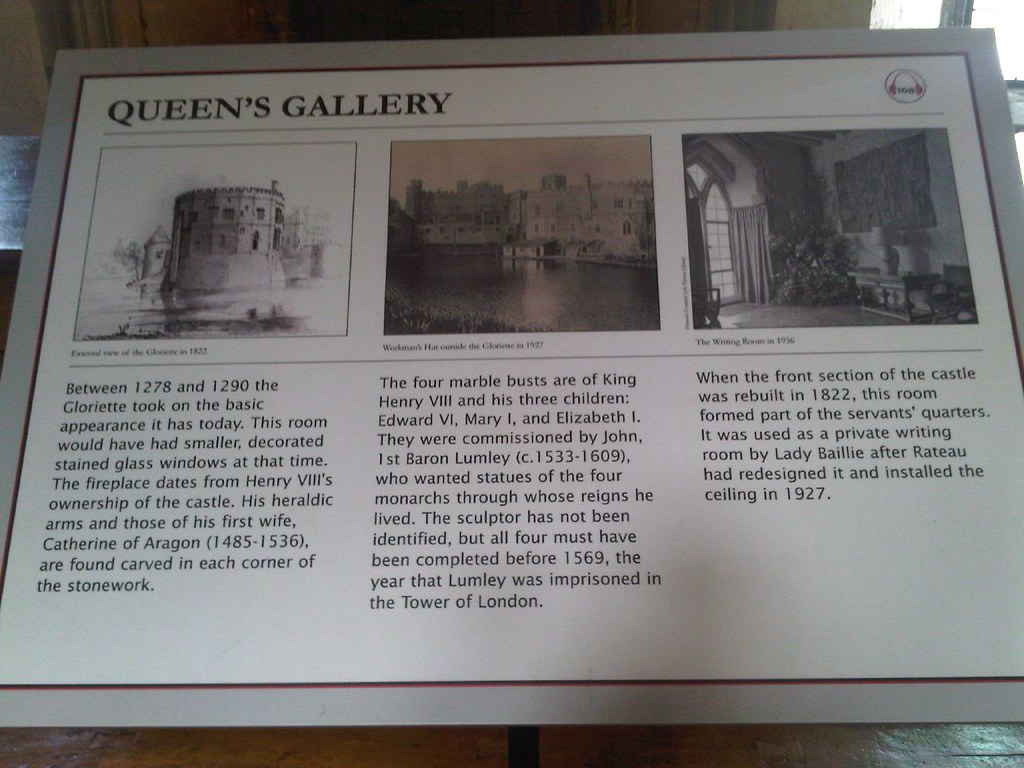The museum placard titled "Queen's Gallery" prominently displays its name in bold text on the top left-hand corner and features a headphones icon in the top right, indicating audio tour compatibility. The placard, angled slightly forward, showcases three images arranged in columns, each accompanied by a title and a paragraph of descriptive text. The images, rendered in black and white or sepia tones, depict different aspects of historical architecture and interiors. The first image likely portrays an exterior view of a castle, highlighting elements such as smaller, decorative stained glass windows dating back to the era between 1278 and 1290. The second image shows a lakeside view with a castle, emphasizing a fireplace from Henry VIII's ownership, featuring heraldic arms of Henry VIII and Catherine of Aragon. The third image captures the interior of what might be the Queen's Gallery itself, elaborating on four marble busts of King Henry VIII and his children, commissioned by John I Baron Lumley, installed before 1569. The text under the final image details the room's transformation into part of the servants' quarters in 1822 and later its redesign into a private writing room by Lady Bollie in 1927. Background objects are faintly visible at the corners of the close-up shot, adding context to the museum environment.